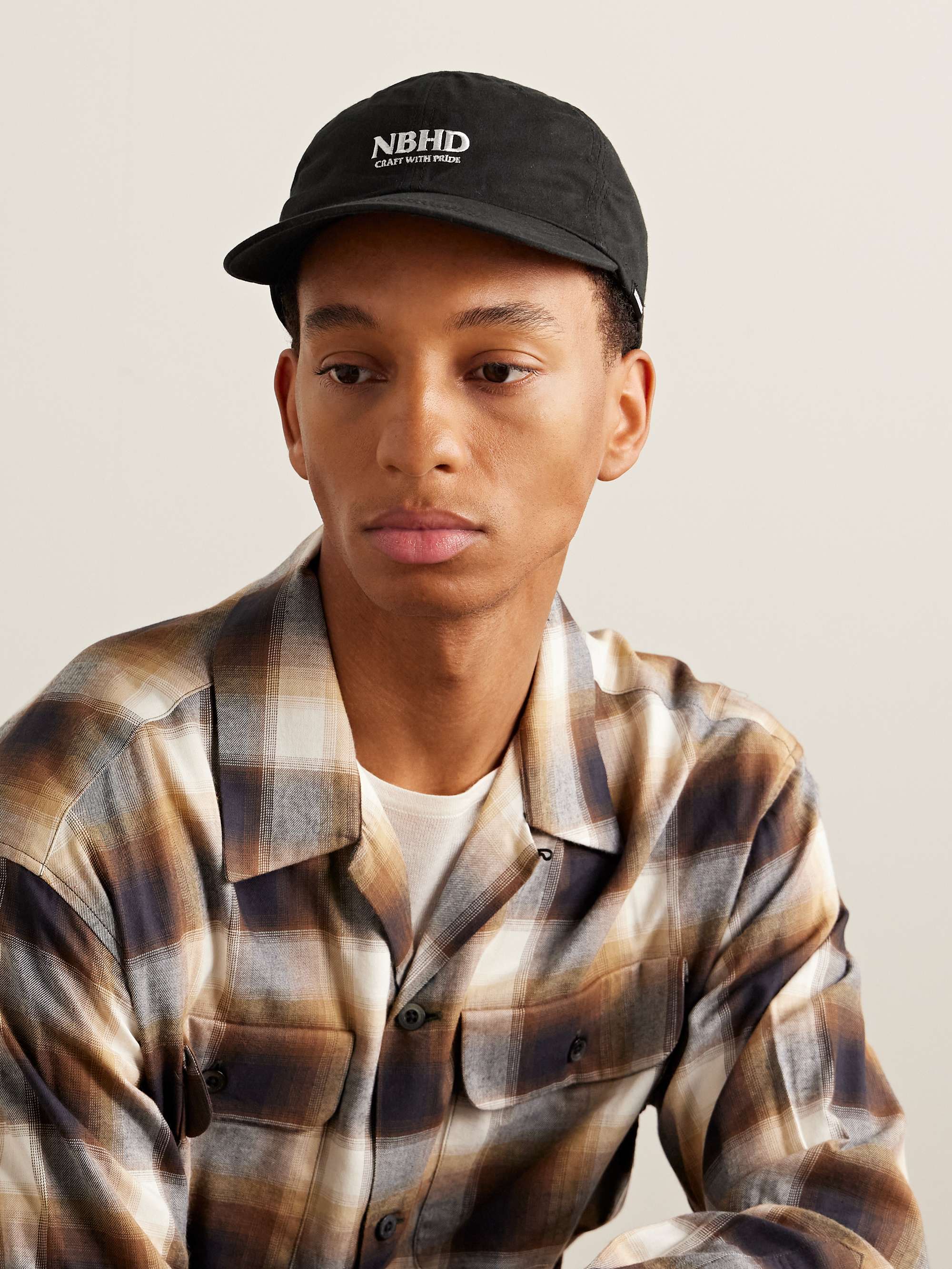In this up-close photograph, we see a young African-American male, likely between 17 and 21 years old, with a light to medium complexion, dark eyes, and red lips. He is wearing a black baseball cap with the letters "NBHD" on it. His attire includes a white T-shirt underneath a buttoned-up flannel shirt featuring a checkered pattern of browns, maroon, white, and hints of yellowish-orange. The flannel shirt has two large front pockets and is mostly buttoned save for the top button, revealing the white T-shirt beneath. He has a very thin face, prominent cheekbones, and a noticeable Adam's apple. The backdrop is a light gray or cream color, and he is staring directly at the camera, capturing a striking and engaging image.